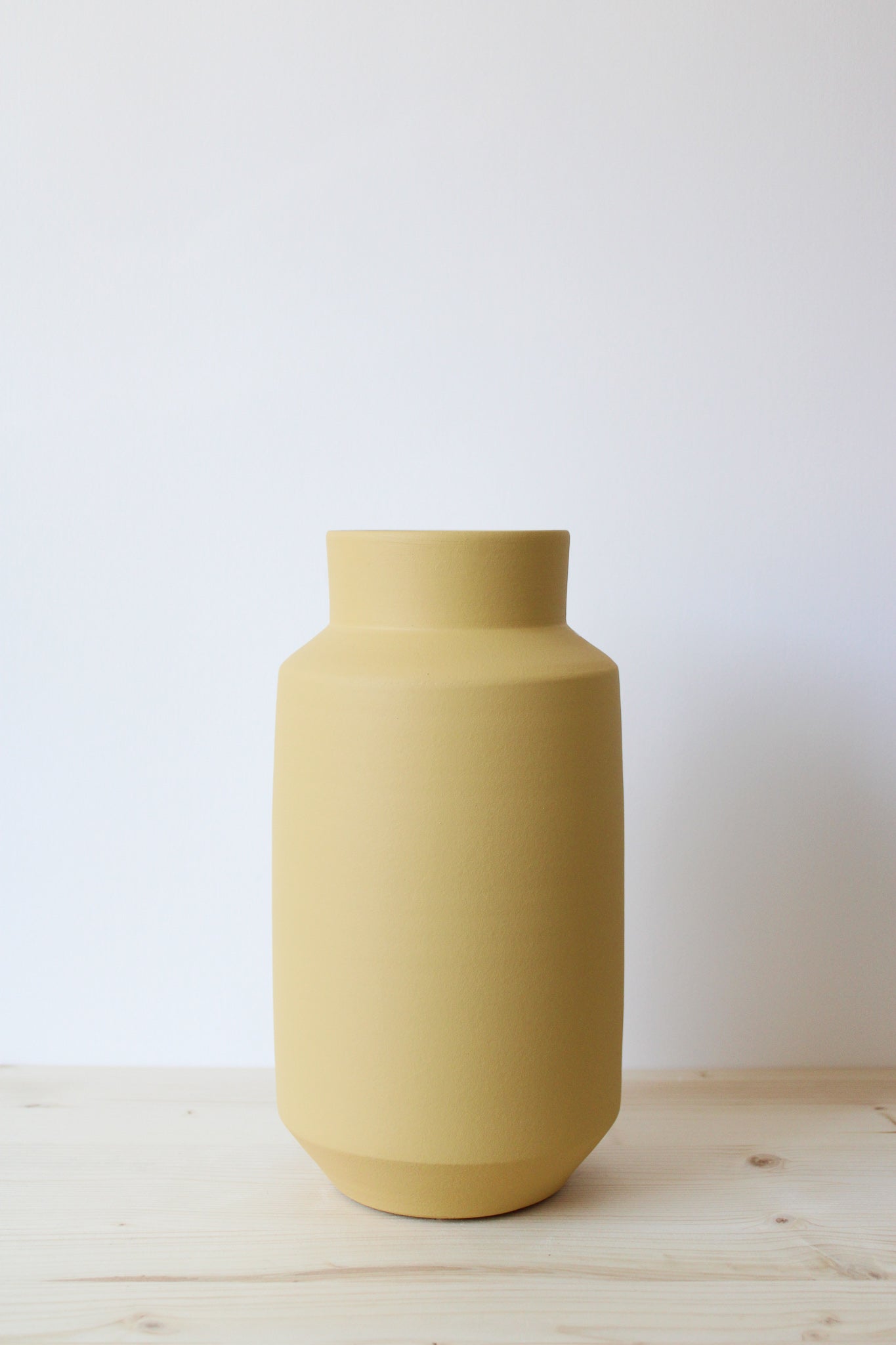This is a detailed colour photograph of a muted ochre yellow ceramic vase, which has a cylindrical shape with a slightly narrower top and a subtle inward curve at the bottom. The vase features a small lip at the very top. It appears handmade, likely formed on a potter's wheel, emphasizing its simple yet elegant design with no additional decorations or colors, reminiscent of something a student might create in an art class. The vase is unglazed, giving it a matte finish that absorbs light rather than reflecting it. It is placed on a pale, unvarnished wooden surface, possibly pinewood, revealing visible grains and slight indentations. The background is a very pale grey, almost white, with a distinct shadow on the right-hand side, suggesting that the light source is coming from the left, casting a soft, even illumination across the scene. No other objects are present in the photograph, enhancing the focus on the vase.